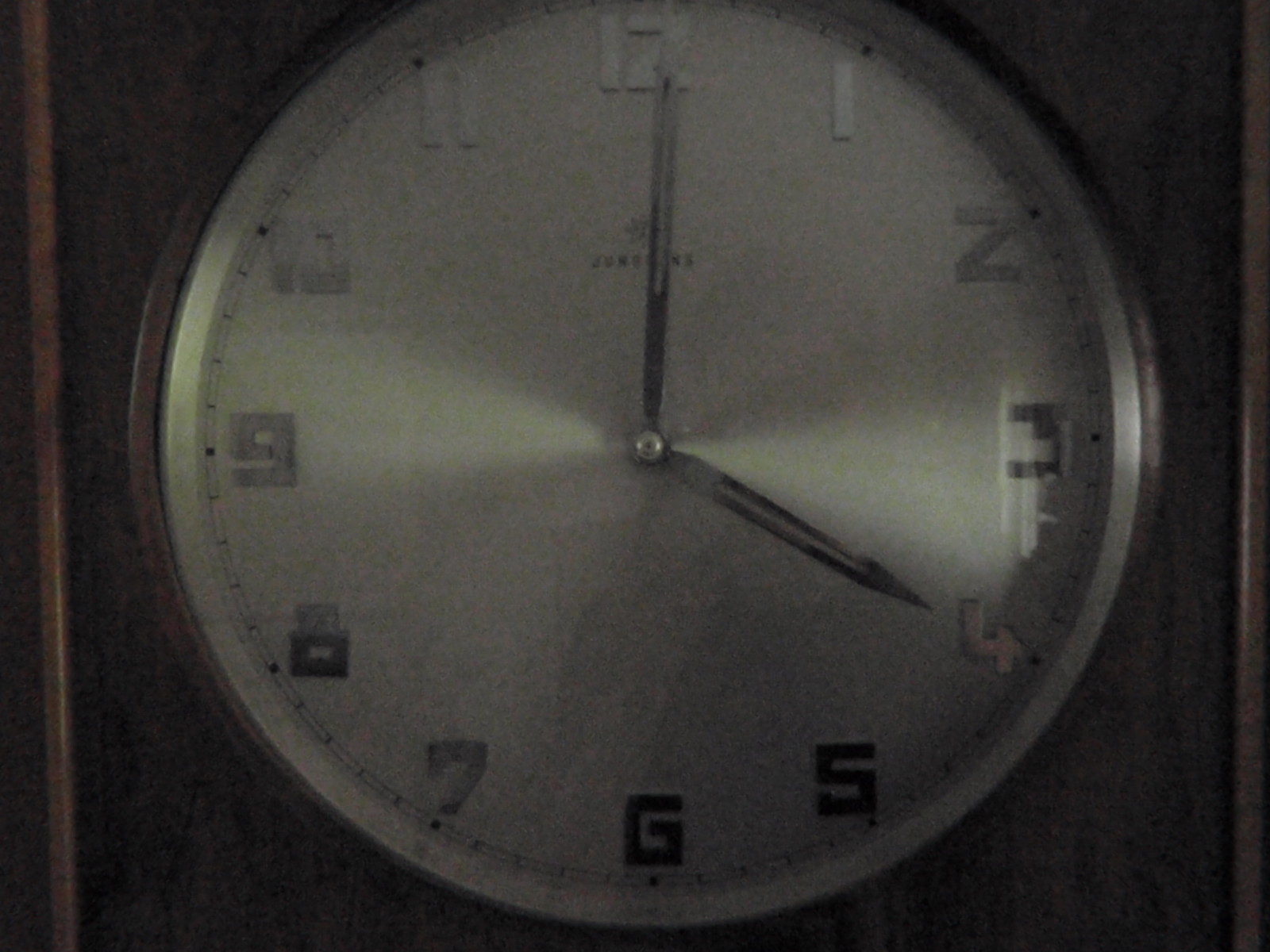This color photograph captures a close-up view of a round clock in a dimly lit setting. The clock's housing is made of dark brown wood with some lighter brown accents, enveloping a white clock face. The face is illuminated primarily at the nine and the three positions, emphasizing these areas in an otherwise shadowy image. The clock’s face features silver, blocky numbers paired with black dots at each numeral and thin hashes marking the minutes in between.

At the center of the clock, a silver pin secures delicate, silver rectangular hands, with the minute hand positioned just past twelve and the hour hand on four. These hands appear thin yet robust, giving the clock a precise and elegant appearance. Although the manufacturer's name is situated between the minute hand and the twelve o'clock position, it is obscured and blurred, making it difficult to discern.

The photograph has a slightly grainy texture and intensely focuses on the clock, occupying nearly the entire frame. There are subtle shadows and hints of light around the edges of the clock, contributing to its dark and somewhat mysterious ambiance. The wood paneling surrounding the clock face provides a sturdy and classic contrast to the sleek, metallic intricacies of the numbers and hands, combining elements of traditional design with a touch of modernity.